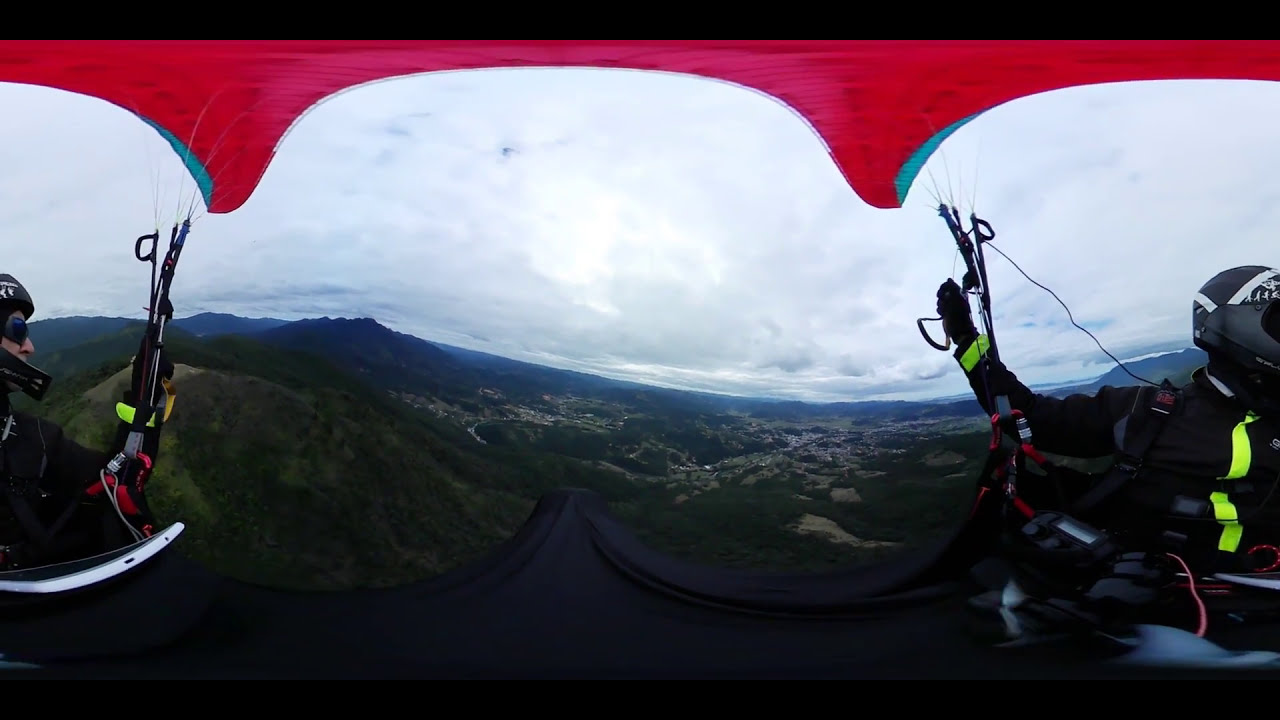This photograph captures the exhilarating moment of two people paragliding under a bright red parachute. The image, shot with a 360-degree camera, offers a comprehensive view of their adventurous flight. The person on the left, wearing a helmet and sunglasses, appears to be looking over at the person on the right, who is adorned with a black and white head covering and a jacket featuring reflective stripes and neon green accents. Both individuals are holding the steering cords of the parachute, navigating their flight.

They are thousands of feet above a green, lush valley, eye-level with the rugged peaks of the surrounding mountains. The landscape below is a mix of rocky terrain and verdant areas with trees and bushes. In the distance, a cloudy sky hovers above a small town nestled in the valley, along with visible roads and buildings. The unique perspective of the 360 camera lens adds a slight warp to the edges, further emphasizing the vastness and splendor of their high-altitude adventure.